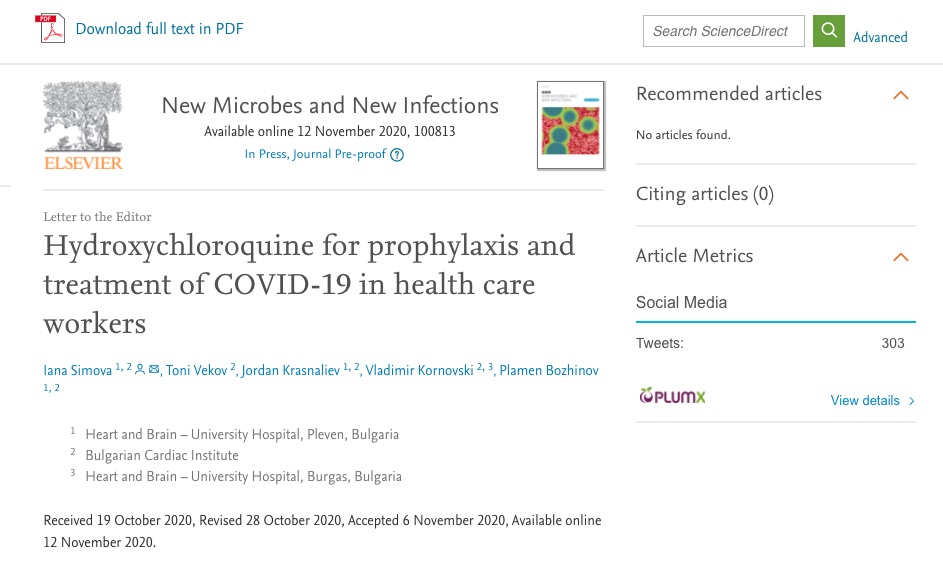The image is a screenshot of the ScienceDirect website, specifically displaying a detailed summary of a scientific article titled "New Microbes and New Infections." The article focuses on the use of hydroxychloroquine for prophylaxis and treatment of COVID-19 in healthcare workers. This study highlights the potential application of the chemical in mitigating the effects of the virus among those on the front lines.

The website's interface is visually structured with a clean white background. In the top left corner, blue text reads "Download Full Text in PDF" adjacent to the Adobe PDF logo. On the top right, a search bar labeled "Search ScienceDirect" is accompanied by a green box with a white magnifying glass icon, facilitating site navigation.

Centrally, the page is dominated by details about the article. The title "New Microbes and New Infections" is prominently displayed, followed by the publication date—12 November 2020. Descriptive text below the title summarizes the study and offers links to the authors and relevant sources, thus providing additional context and avenues for further exploration.

On the right side of the page, a vertical sidebar features a variety of clickable links directing users to recommended articles, article metrics, and other sections of the website. This sidebar enhances user engagement by offering more content related to the featured article.